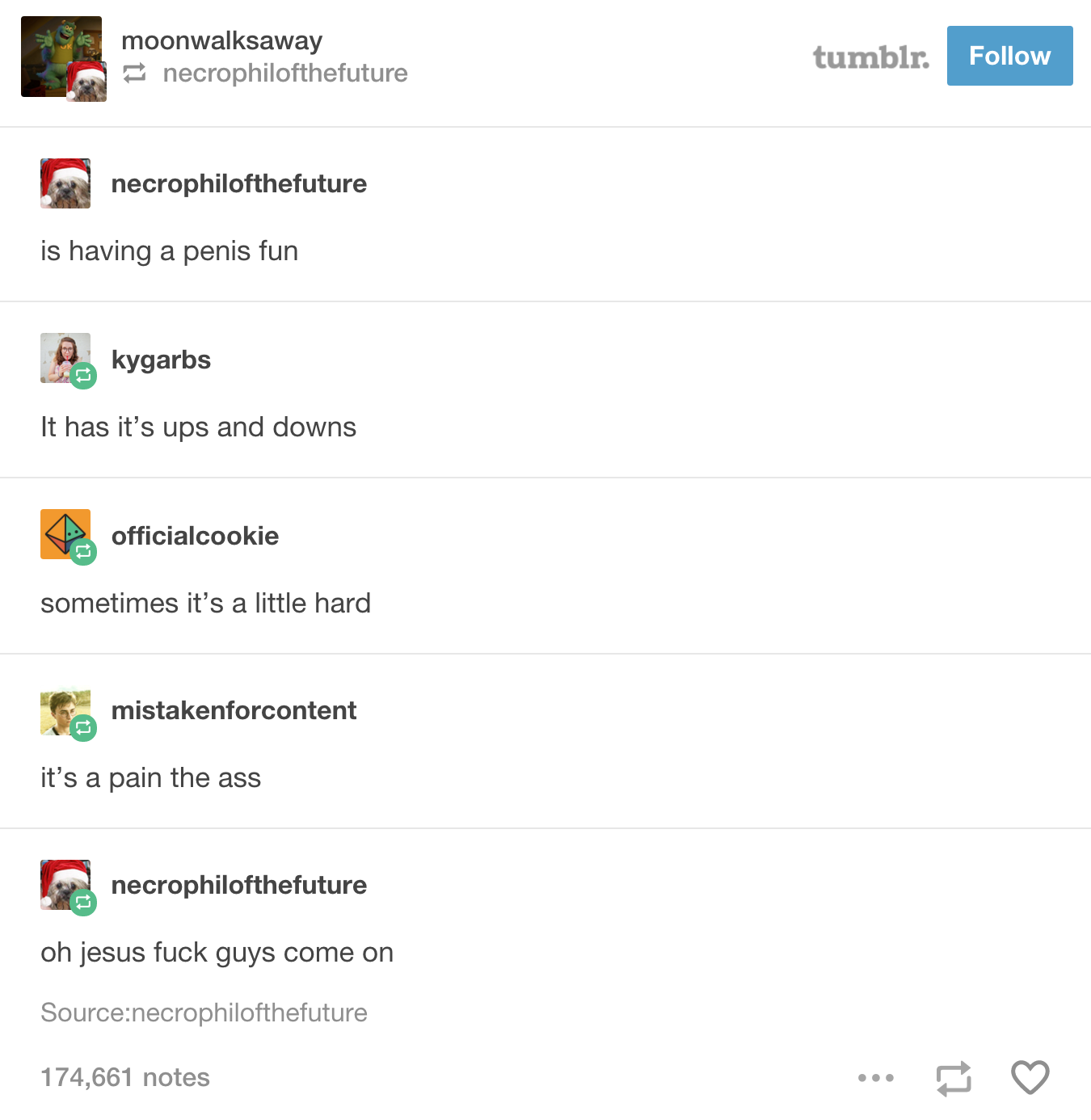Screenshot of a Tumblr page showing a conversation thread:

- On the left-hand side, there's an image of a green alien next to a dog wearing a Santa hat. Overlaid in black text is "moon walks away."
- This is a reply to the user "necrophil of the future," which reads "ew."
- On the right, the page features Tumblr's grey logo and a light blue circle with the word "foul" in white.
- Below the logo, the user "necrophil of the future" asks, "is having a penis fun?"
- A user named "Kai Garbs" responds, "it's ups and downs."
- Another user, "cookie, official cookie," adds a comment: "sometimes it's a little harder than mistaken for content, it's a pain in the ass."
- "necrophil of the future" reacts again with, "oh Jesus fuck guys, come on."
- The source of the post is credited to "necrophil of the future," with 174,661 notes counted.
- In the bottom right corner, there are three dots representing more options and the outline of a heart, indicating the "like" feature on Tumblr.

The screenshot captures the chaotic and somewhat nonsensical nature of this Tumblr discussion, highlighting why some users find the platform frustrating.